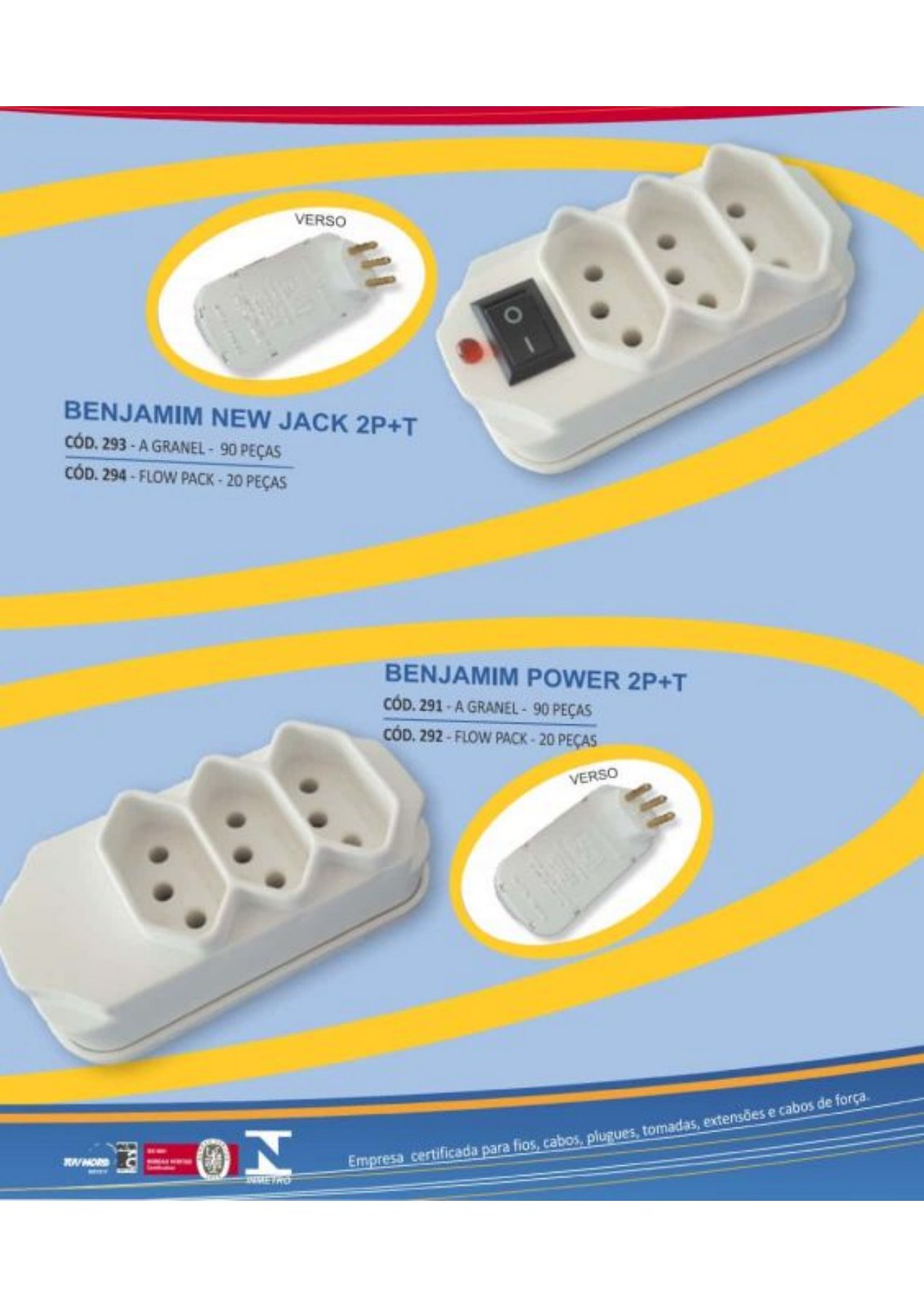The image depicts a detailed informational poster set against a pale blue background. The design features several yellow ovals highlighting the core components being advertised. At the top, a yellow hat-like shape is seen, resembling the upper part of an oval, beneath which are illustrated various power-related devices. The primary focus is a sophisticated power outlet with a switch positioned on top and a jack highlighted inside a yellow circle, surrounded by a white interior. The text "Verso" is clearly visible above the outlet. To the right, shown prominently, are power adapters or strips with different configurations, each featuring three circular prongs, designed in a slim style divergent from conventional American designs. Directly below, labeled in blue print, are the descriptions "Benjamin New Jack 2P plus T" and "Benjamin Power 2P plus T" with accompanying codes. Notably, the upper device includes a red LED and a power switch, absent in the lower model. Additional text at the bottom of the poster, written in Portuguese, states, "empresa certificada por afios, cabos, plugges, tomates, extendios, y cabos de forca," indicating certification and compliance with standards for various electrical products.